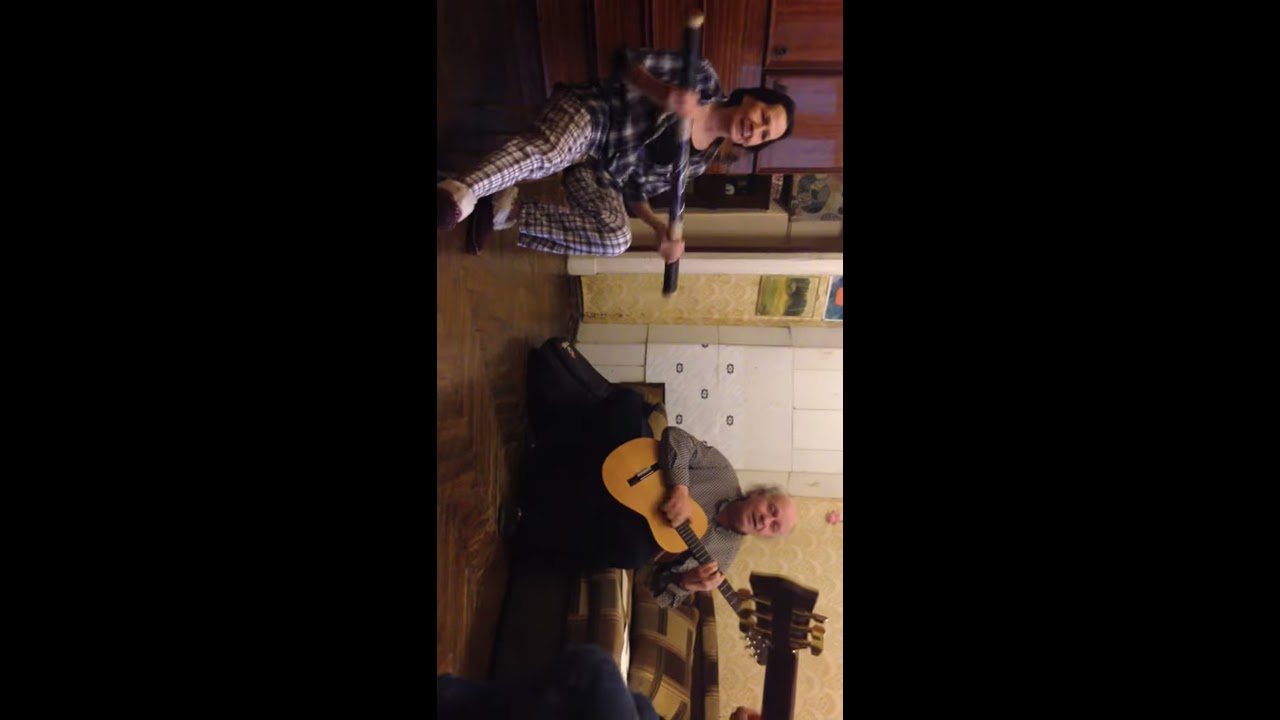This photograph, rotated 90 degrees to the right and flanked by two vertical black strips, depicts an intimate indoor scene. Centered in the image are an older man and a woman, both immersed in music. The man, seated on a brown sofa, wears a long-sleeved gray shirt and strums an acoustic guitar, his mouth slightly open in song. To his left, on the wooden floor, sits a woman in a blue plaid shirt, plaid sleep pants, and slippers, holding a cylindrical rainmaker. A third person is partially visible on the right side of the image, identifiable only by the back of their knee and the handle of their guitar. The room features a brown wooden floor, and the setting appears to be a cozy living room bathed in various hues of black, brown, light brown, gray, tan, gold, blue, orange, and green. The scene suggests a casual, perhaps impromptu, musical gathering.